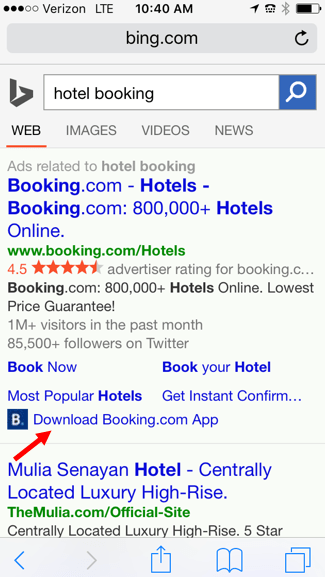Screenshot of a Smartphone Displaying a Bing.com Search Page

The image is a screenshot captured on a smartphone, showcasing the Bing search engine interface. At the top of the screen, the status bar is visible, indicating the phone's signal strength with several bars, a Verizon LTE network connection, the current time centered, and various icons on the right, including the battery level, Bluetooth status, and location services icon.

Below the status bar, the web browser's address bar clearly displays "bing.com" with a refresh icon adjacent to it. Directly underneath is the Bing search bar. The left side of the search bar features the Bing logo, and the right side contains a search query input area that currently reads "hotel booking" next to a blue search button.

Under the search bar, there are four distinct tabs for categorizing search results: "Web," "Images," "Videos," and "News." The "Web" tab is highlighted in bold and underlined in red, indicating that it's the active tab showing web page results.

The main portion of the screenshot displays search results for "hotel booking." The first result is an advertisement for booking.com, promoting 800,000 hotels online. This ad includes a green URL link, a 4.5-star rating, a brief description, and various sub-links for additional information.

The subsequent result features Mulia Senyin Hotel, described as a centrally located luxury high-rise. Similar to the first result, this entry includes a URL and the beginning of a descriptive caption.

Additionally, a notable red arrow points to a link encouraging users to "download booking.com app," with the booking.com logo positioned beside it, suggesting this area is of particular interest for further action.